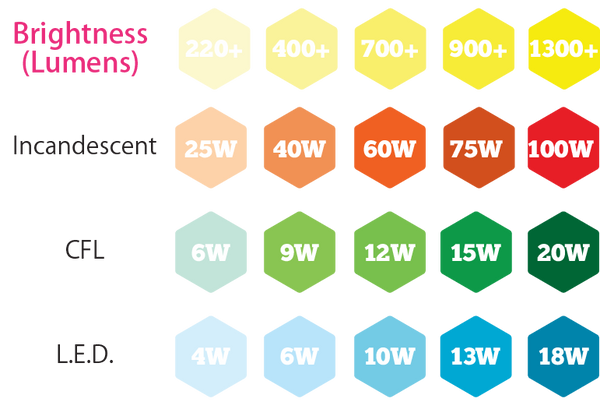The image features a detailed chart depicting different types of light bulbs represented in rows and columns of hexagons. The top left corner of the chart is labeled "Brightness (lumens)" in dark pink text, and adjacent to this label is a row of five hexagons transitioning from light gray to vivid yellow, each marked with increasing lumen values: "220+", "400+", "700+", "900+", and "1300+".

Below this, there are three additional rows labeled "Incandescent," "CFL," and "LED," each accompanied by a series of five hexagons in varying colors that indicate wattage. 

- The "Incandescent" row features hexagons colored from pale orange to deep red, labeled with wattages: "25W", "40W", "60W", "75W", and "100W".
- The "CFL" row has hexagons that transition from light green to dark green, marked with "6W", "9W", "12W", "15W", and "20W".
- The "LED" row displays hexagons shading from faint gray to solid blue, denoting "4W", "6W", "10W", "13W", and "18W" respectively.

The consistent transition of colors within each row visually represents increasing brightness or wattages from left to right, creating a comprehensive overview of light bulb types and their corresponding energy outputs.